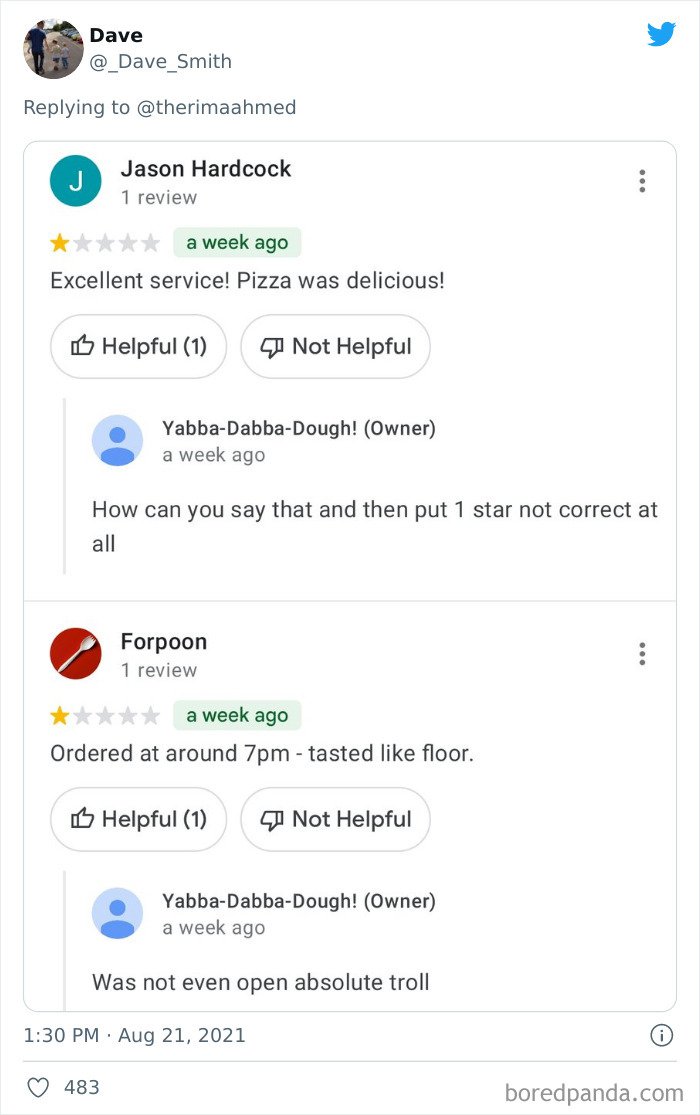This image appears to be a screenshot of a review section on a social media platform. In the upper left corner, there is a small profile picture of a man, accompanied by the handle "Dave" (@Dave_Smith), who is replying to "The Rima Med." A blue bird icon, typical of Twitter, is visible in the upper right corner. Below, there is a highlighted review from Jason Hardik, who has left one review and rated it one star, despite praising the service and food as "excellent" and "delicious." His review was posted a week ago and has options for marking it as "helpful" or "not helpful." The owner, using the name "Yabba Dabba Doe," responded a week ago, expressing confusion and disbelief at the one-star rating.

Further down, another review from "Four Poon," who has also given one review and rated it one star, describes the order made at 7 p.m. as tasting like the floor. This review has also been flagged as either "helpful" or "not helpful." The same owner, "Yabba Dabba Doe," replied a week ago, countering the claim by stating the establishment was not open at that time and calling the review a troll. The timestamp at the bottom of the screenshot reads "1:30 p.m., August 21st, 2021."

This detailed caption captures the content and context of the image with specificity.